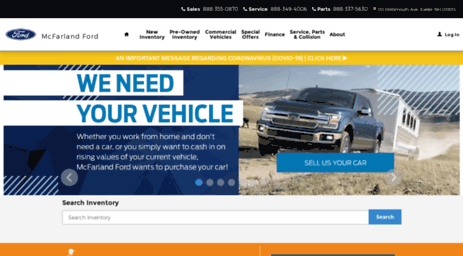This screenshot captures the homepage of the McFarland Ford website, featuring a variety of sections catering to different customer needs. The navigation menu prominently includes links to "New Inventory," "Pre-Owned Inventory," "Commercial Vehicles," "Special Offers," "Financing," "Service Parts and Collisions," and an "About" section. Additionally, there is a login area for user accounts. 

An infographic ad occupies part of the screen, stating: "We need your vehicle. Whether you work from home and don't need a car or you simply want to cash in on the rising values of your current vehicle, McFarland Ford wants to purchase your car." This ad includes an actionable "Sell Us Your Car" button, and arrow buttons for scrolling through more similar advertisements.

Below the ad, a search bar allows users to directly search for specific Ford models within the dealership's inventory. 

The top of the page lists phone numbers for various departments such as sales, service, and parts, providing convenient contact options for customers. Despite some clutter, the site features a compelling image of a Ford vehicle navigating rugged terrain, highlighting the brand’s reliability and durability.